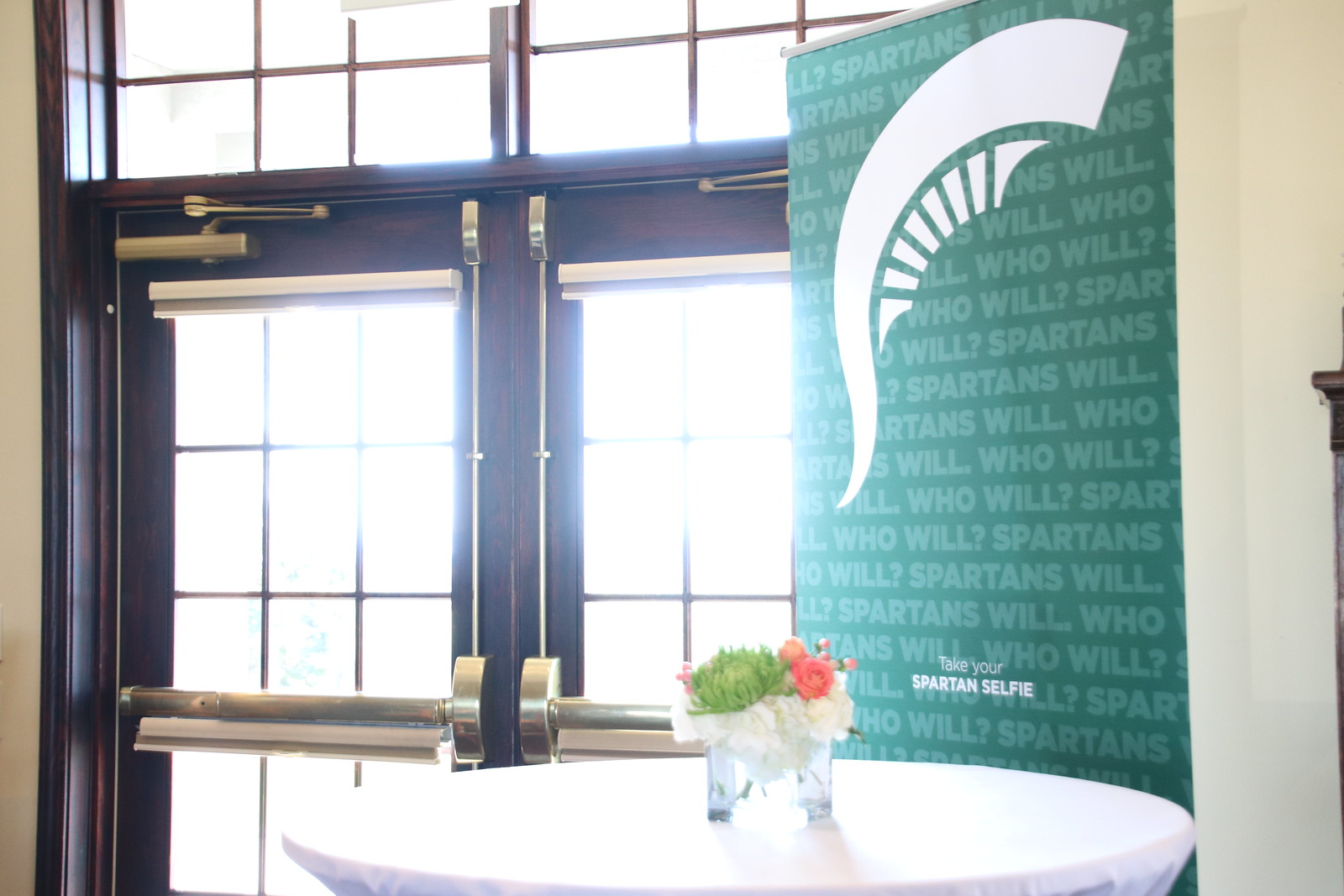The photograph depicts a meticulously arranged white circular table adorned with a thin white tablecloth. Atop the table, two clear vases take center stage—one filled with vibrant pink roses, and the other showcasing lush green plants. The scene is set within a function hall, where sunlight filters through a set of double doors with windows. To the right of the table, a tall, dark green banner prominently features the white silhouette of a Trojan helmet, the top curved part of it discernible. The banner is patterned with the phrase "Spartans Will. Who Will?" in lighter green text repeated throughout. At the very bottom of the banner, smaller text invites attendees to "take your Spartan selfie." The overall ambiance is illuminated by the natural light streaming through the closed doors in the background, adding a warm glow to the setup.